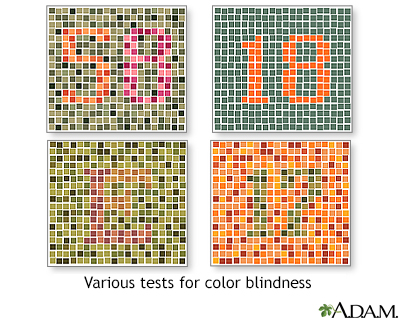The image features a series of four colorblindness test squares, each showcasing a different figure made up of small colored squares that blend into varying backgrounds. The squares are arranged in a grid with a completely white background. The top-left square features the number 58, while the top-right displays the number 18 against a green background with orange numerals. The bottom-left square depicts the letter E, framed by a pattern of varying shades of green checkers. Lastly, the bottom-right square shows the number 17, composed of small orange and red checkers. Below the grid, text reads "various tests for colorblindness," followed by the name "Adam." The test challenges viewers to discern the figures, which can be difficult for those who are colorblind.